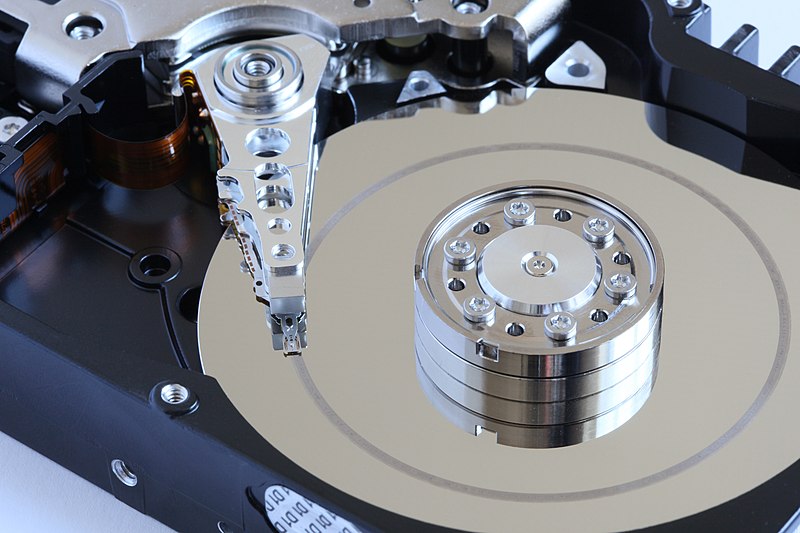This detailed image showcases the intricate internal components of a hard drive. At the center lies a silver platter, which serves as the primary data storage area. Surrounding the platter are various screws that fasten the components together securely. Notably, magnets are in place to position and guide the reading arm precisely. The reading arm itself is equipped with several rings and perforations, indicating its complex mechanical design. The hard drive is encased in a black plastic body, which includes additional securing screws and printed text, likely detailing specifications or instructions. This visual dissection offers a comprehensive look at the hard drive's inner workings, revealing the spindle, reading arm, magnets, and supportive casing.